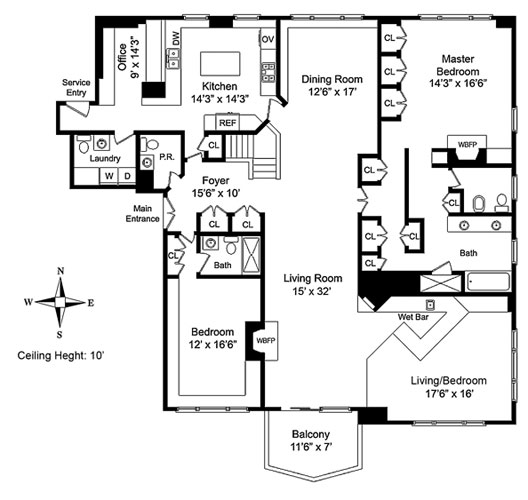This detailed architectural drawing illustrates the floor plan of a residence with meticulous measurements and room placements. Upon entering the main entrance, you are greeted by a foyer. To the right of the foyer, there is a bedroom measuring 12 feet by 16.5 feet, complete with an en-suite bath and a closet. Moving left from the entryway, you'll find a spacious 14 by 14 feet kitchen designed with a center island. Adjacent to the kitchen is a 9 by 14 feet office, which features an external service entrance.

Directly opposite the office is a laundry room equipped with a washer, dryer, and a toilet. From the foyer, a stairway is positioned on the left side. Proceeding forward, the floor plan opens up to a 12 by 17 feet dining room on the left and a 15 by 32 feet living room to the right, which includes an inviting fireplace. The living room also opens up to an 11.5 by 7 feet balcony, offering outdoor space.

Additionally, there is another generously sized room measuring 17 feet 6 inches by 16 feet that can serve as a secondary living area or bedroom, and it features a wet bar for added convenience. The master suite includes a master bedroom measuring 14 feet 3 inches by 16 feet 6 inches, with multiple closets in the vicinity. The master bath is well-appointed with a shower, tub, and toilet.

The architectural drawing also indicates the cardinal directions with arrows pointing north, east, west, and south, and notes a ceiling height of 10 feet in the legend.